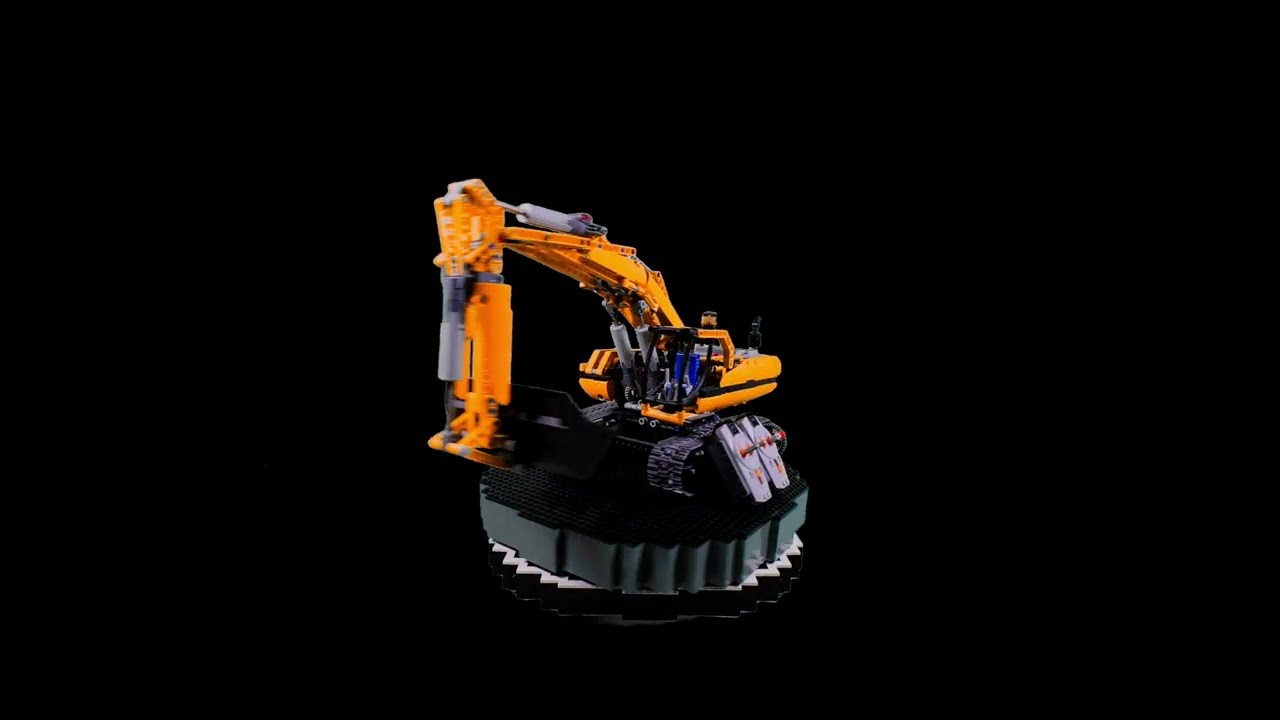The photograph features a detailed model of a toy construction crane, prominently highlighted against a pitch-black background that provides no additional context. The crane itself is predominantly orange, though it has been described variably as yellow, and features a raised boom that is equipped with an extending arm, ending with a vertically hanging component. The vehicle is mounted on tank-like black treads, which convey a sense of rugged, all-terrain capability.

Attached to the crane model is a gray platform, textured like a LEGO pedestal, complete with rivets. There is a small figure in the cockpit, suggesting the crane is indeed a toy. Remote control elements are also present, further indicating its status as a toy.

The composition of the photograph centers the model both horizontally and vertically. The crane's detailed mechanisms, including multiple gray mechanical pieces, reinforce its intricate design, making it look more like an industrial vehicle. Despite varied descriptions, the overall impression remains consistent: a brightly colored, meticulously crafted model crane set against an utterly black backdrop.